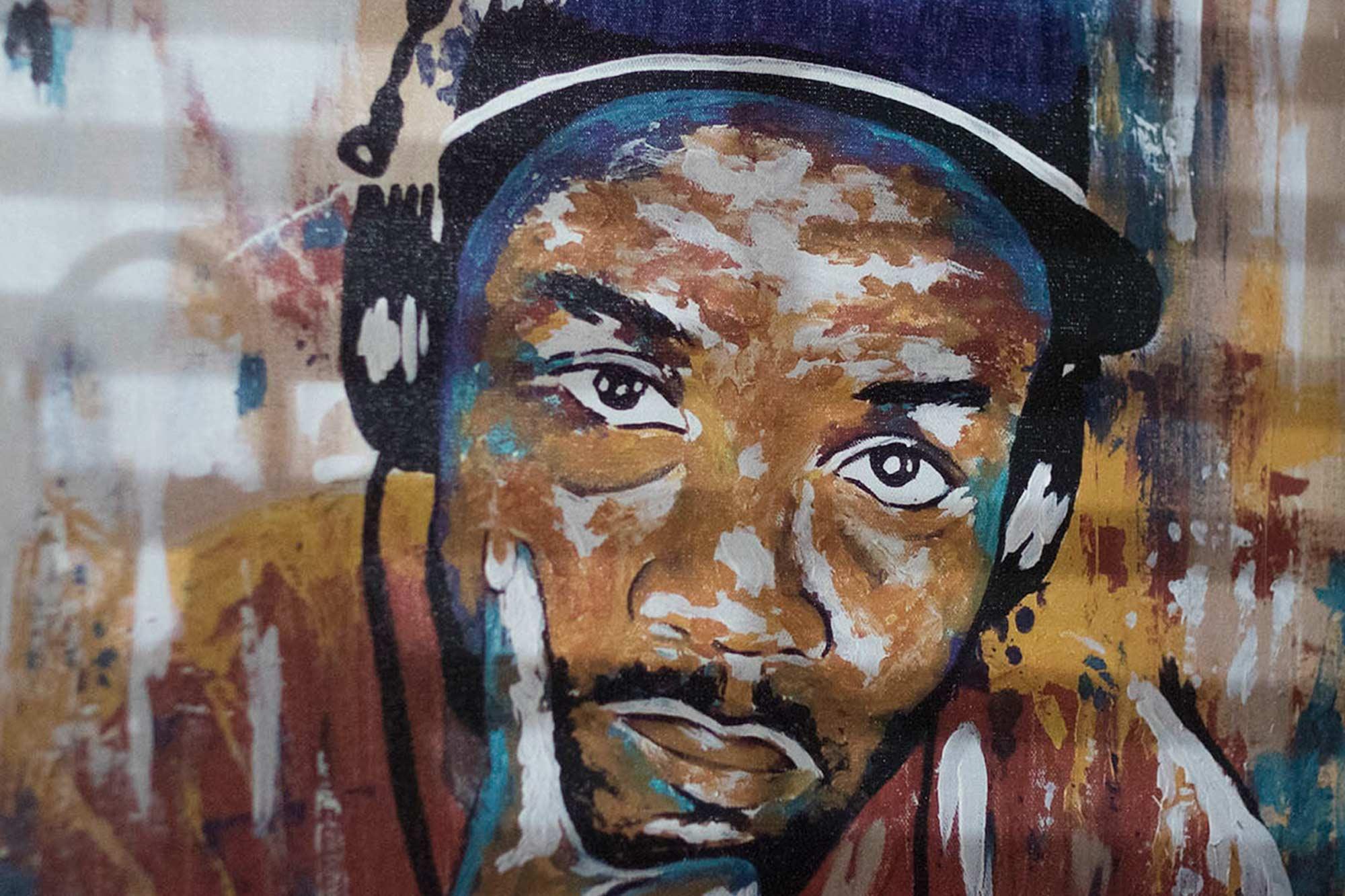The image is a horizontally rectangular, abstract painting that vividly captures the likeness of a young African American man. The painter employs dynamic, splashing strokes of various colors, lending a spotty and non-solid finish to the artwork. The man's light brown face is accentuated with white streaks, especially on his forehead and beneath his eyes, and framed by a short black beard and mustache. His mouth is slightly open, revealing a glimpse of his tongue through his lips.

He dons a navy blue baseball cap adorned with a white ribbon and wears over-the-ear black headphones with visible wires. His left hand is thoughtfully resting on his face, with his thumb or index finger touching his cheek. His gaze is neutral, neither smiling nor frowning, directed straight ahead. The composition extends into a background filled with aggressive streaks and splashes of paint, including reds, yellows, aqua blues, and subtle gray and white stripes. The man's shirt is a burgundy-red hue, blending seamlessly with the vivid, multicolored backdrop that emphasizes the abstract, energetic style of the piece.